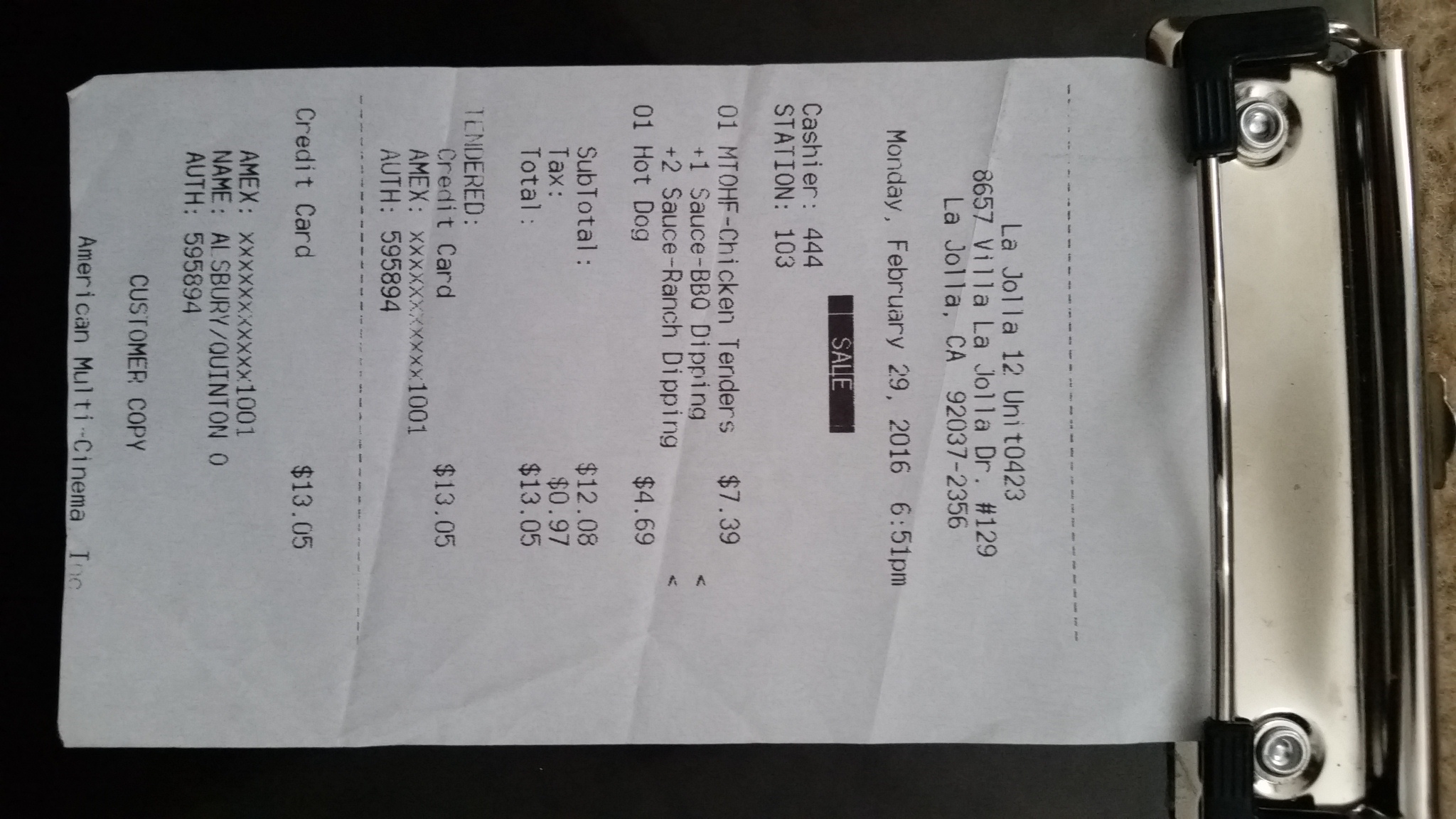In the image, there is a white receipt secured by a small metal arm. The receipt details a purchase made at La Jolla 12, located at 8657 Villa La Jolla Drive, Unit 0423 #129, La Jolla, California. The transaction occurred on Monday, February 29, 2016, at 6:51 PM. The cashier, identified by number 444, operated at station 103. The items purchased include chicken tenders priced at $7.39 and a hot dog for $4.69. The subtotal for these items is $12.08, with an additional tax of $0.97, making the total $13.05, which was paid using a credit card. At the bottom of the receipt, it is marked as the customer copy from American Multi-Cinema.